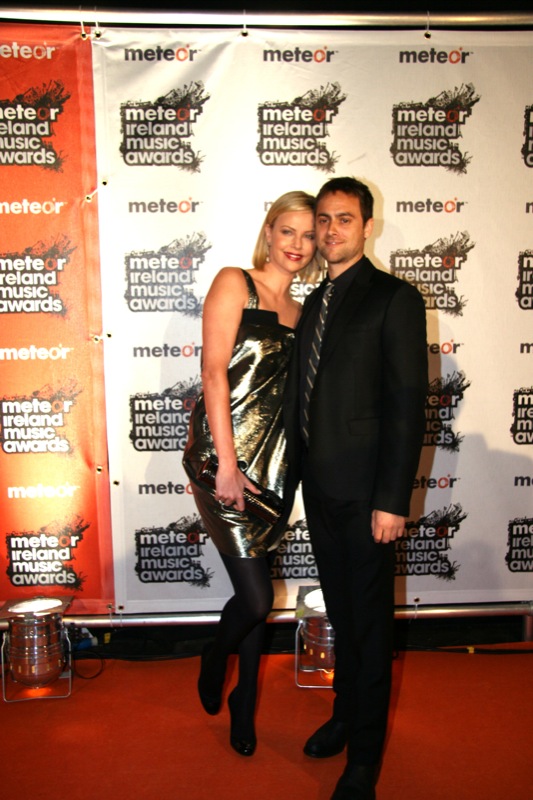The photograph features a well-dressed couple at the Meteor Ireland Music Awards event, standing on a red carpet. The woman, positioned on the left, is wearing a shimmering metallic gold dress that reflects the light, adding a touch of glamour. Her short blonde hair falls just to her neckline, and she completes her outfit with black pantyhose and heels. She carries a small purse or satchel and has a leg slightly raised, leaning towards the man beside her. She sports red lipstick and is smiling while looking to the left. The man, to her right, is dressed in a black suit with a matching shirt and pants. His tie is black with silver accents, and he has short black hair. He, too, is looking to the left, smiling, with his arm down by his side. Both individuals are Caucasian.

Behind them hangs a white banner with the Meteor Ireland Music Awards logo repeated in a grid pattern, featuring white text on a black background and sporadically incorporating the word “Meteor” in black with a red "O". Additionally, an orange banner with the same logos is visible to the left. Small spotlights on the floor illuminate the scene, pointed upwards towards the couple, adding to the celebratory atmosphere. A few drums are also placed on the red carpet near the backdrop.